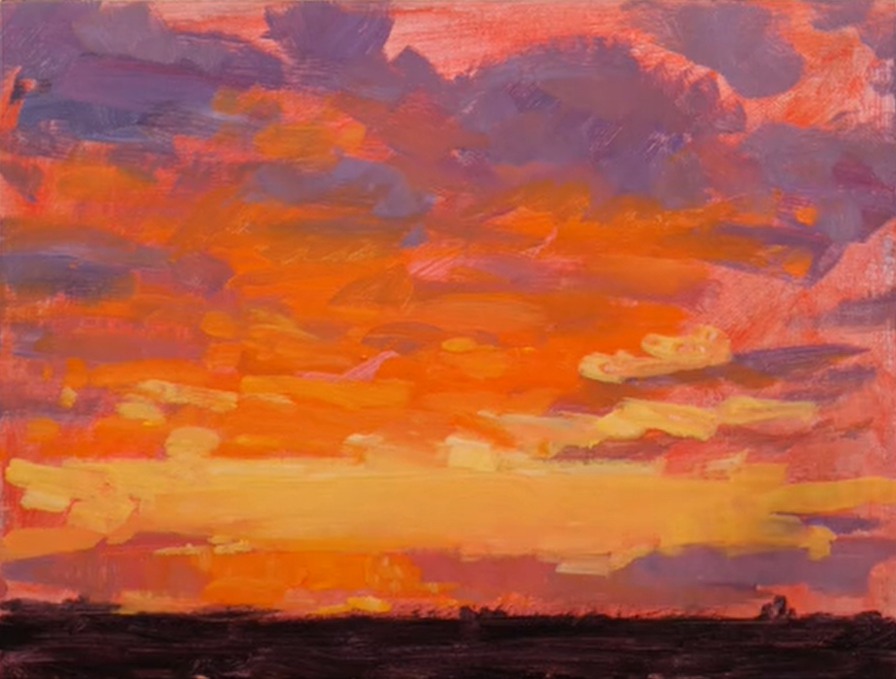The image beautifully captured in the painting is a vivid and expressive depiction of a sunset sky created using oil colors. Brushstrokes sweep horizontally across the canvas, showcasing a spectrum of colors that transition smoothly from bottom to top. At the base of the painting, a dark grayish-black land serves as a stark background, juxtaposing the vibrant sky above. This horizon is almost entirely black, providing a grounding element beneath the colorful expanse.

The sky itself is a harmonious blend of clouds in various hues. Near the horizon, clouds glow with warm amber and yellow tones, transitioning to rich oranges and finally ascending to bluish-purple at the upper reaches of the canvas. These clouds are rendered with textured brushstrokes, adding depth and movement to the scene. Amidst this array, hints of white punctuate the clouds, adding highlights that suggest the sun’s rays piercing through.

The backdrop sky behind the cloud formations is a delicate amalgamation of pink and purple shades, enhancing the overall warmth and tranquility of the painting. An orange, roundish area near the horizon symbolizes the sun in its final moments before nightfall, casting a brilliant light that tints the surrounding clouds with golden hues. This evocative representation encapsulates the serene beauty of a sunset, with each brushstroke and color carefully chosen to convey the artist's vision of a majestic evening sky.